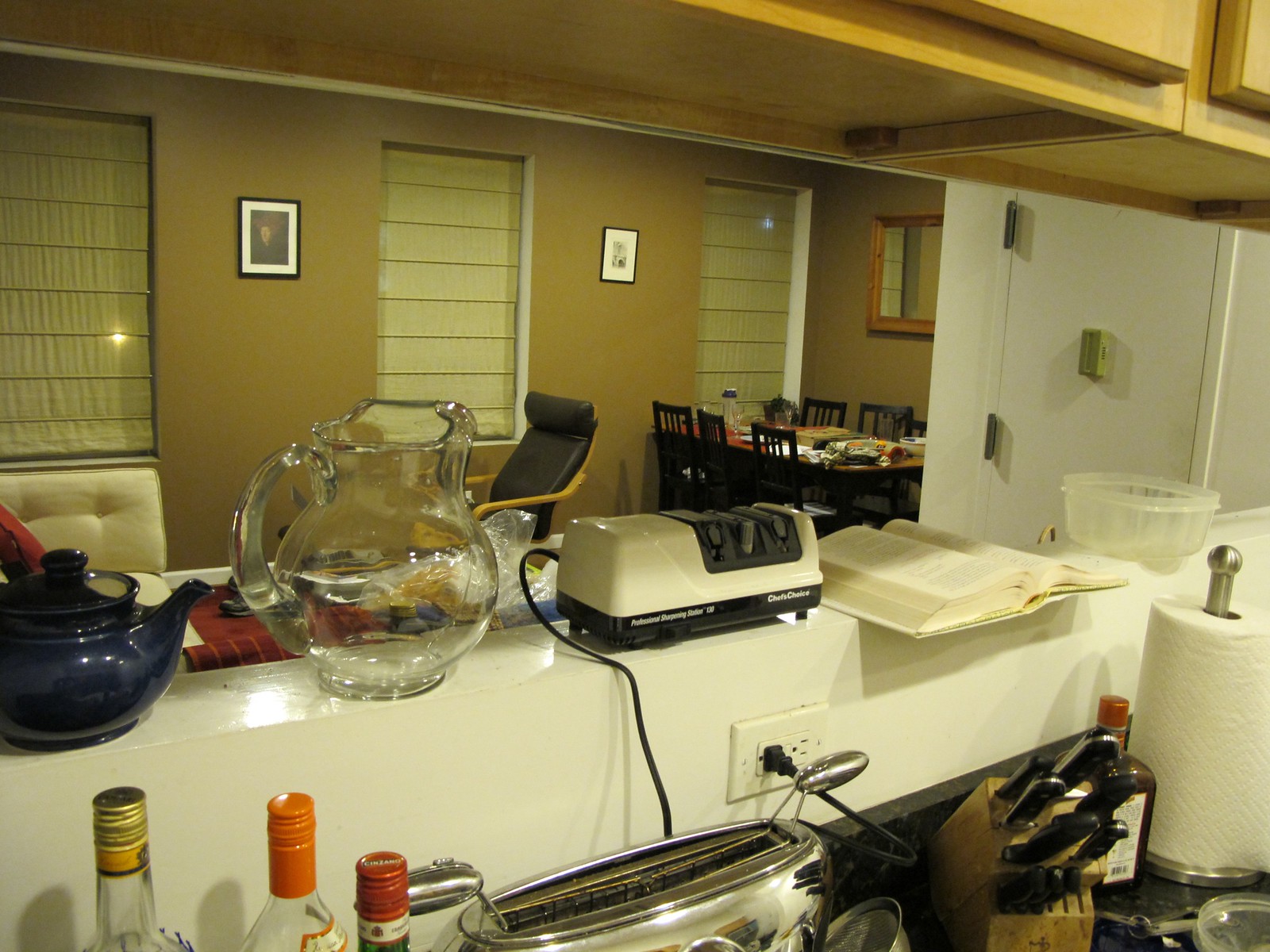The image captures a cozy, lived-in kitchen, likely part of a home. The photograph is taken from within the kitchen, offering a view through an opening in the wall into an adjacent room. 

In the foreground, a well-used wooden table with six chairs stands as a central feature. The table is cluttered with an assortment of items, hinting at daily activities and a bustling household. The walls, painted in a brown taupe color, provide a warm backdrop to the scene.

Three windows dressed in khaki-green-brown coverings allow natural light to filter into the space. The decor includes two framed pictures hanging on the wall, adding a personal touch. 

On the ledge of the opening between the kitchen and the adjacent room, a variety of objects are neatly placed from left to right: a charming blue teapot with a lid, a clear glass pitcher, an unidentified appliance with a cord, an open book, and a transparent plastic container.

In the very foreground, partially visible on the kitchen counter, there are three bottles, likely containing liquor, their lids glinting in the light. An unidentifiable silver appliance with twin handles stands next to a wooden block filled with black-handled knives. Another bottle with a red lid sits alongside a silver paper towel holder, which holds a roll of white paper towels.

Dominating the background, a white wall features a door with visible hinges on one side. Brown overhead cabinets or cupboards can be seen at the top, showcasing the underbelly of typical kitchen storage space.